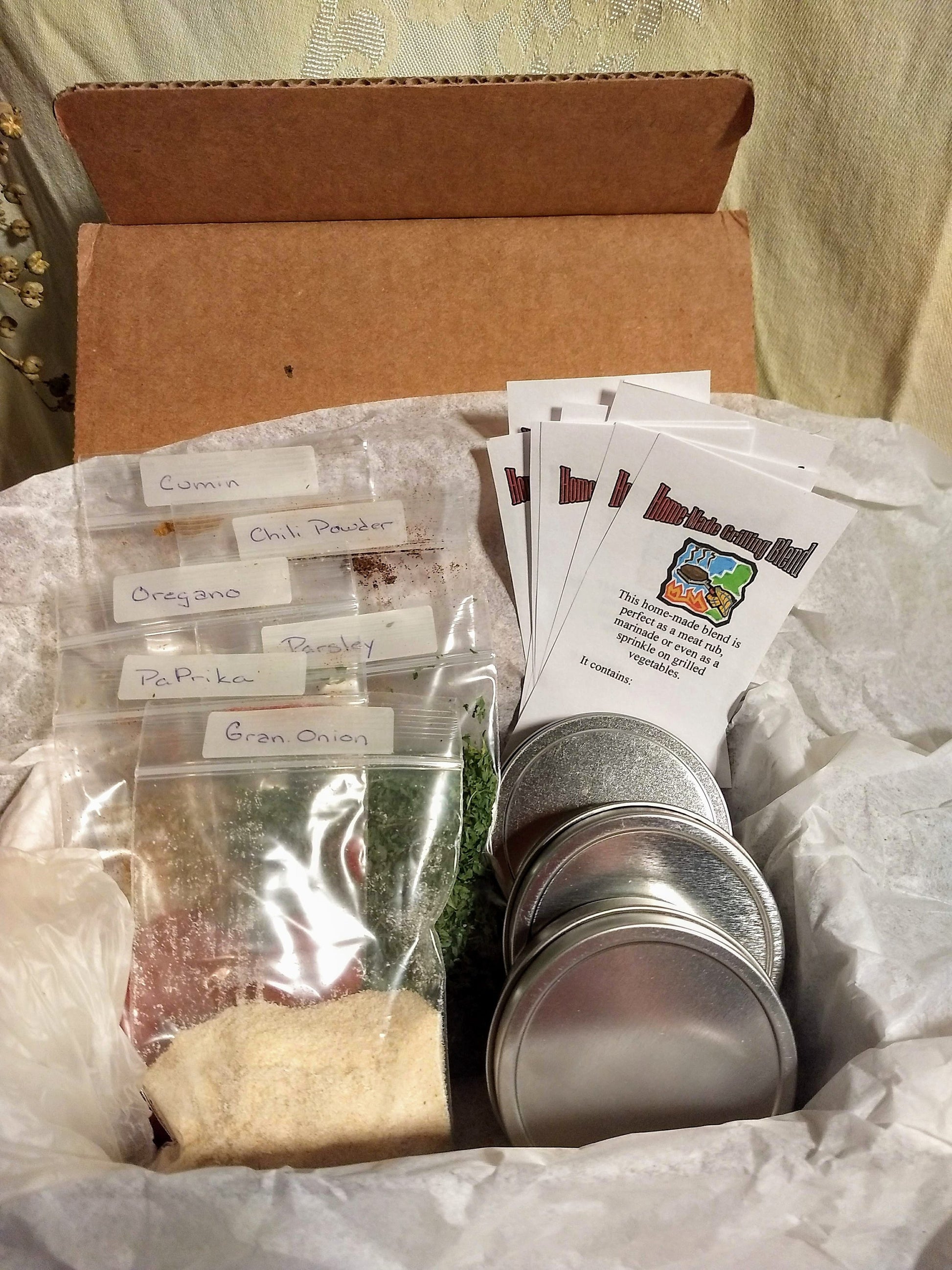Inside a cardboard box lies a delightful assortment of spices and grilling essentials, perfectly organized for an avid cook or grilling enthusiast. The box is lined with white packing paper that cradles several Ziploc baggies filled with various spices on the left and a few polished silver tins on the right. The foremost Ziploc bag contains a white-ish powder labeled "Ground Onion," while behind it, other bags are neatly arranged, bearing labels for spices like paprika, parsley, oregano, chili powder, and cumin.

To the right of these bags are three small, reflective silver tins stacked one behind the other. Further back, adding a touch of information and whimsy, is a stack of six neatly placed flyers. Each flyer bears the heading "Saito Homemade Grilling Blend" in colorful text with a black ink outline and a small cartoon of a person grilling. The pamphlets enthusiastically describe the blend's versatility as a meat rub, marinade, or a seasoning for grilled vegetables. This carefully curated collection of spices and informative pamphlets, wrapped thoughtfully, seems to be a homemade gift box designed to enhance the grilling experience.